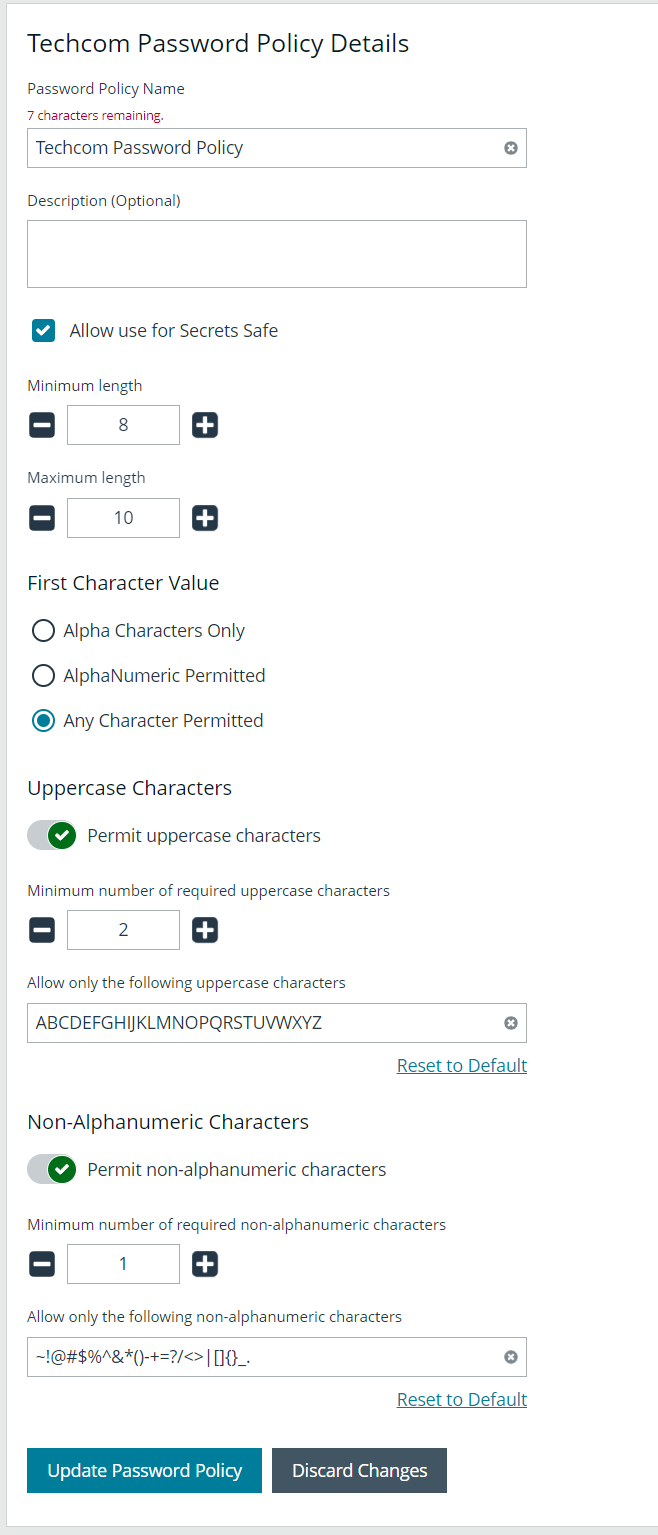### Caption

The image showcases a detailed webpage outlining the TACCOM Password Policy settings. The headline "TACCOM Password Policy Details" is prominently displayed at the top. Below that, a section labeled "Password Policy Name" includes a note in red indicating "seven characters remaining." A search bar below this contains the policy name "TACCOM Password Policy" and features a white X in a gray circle for clearing the entry.

Following the search bar, the page offers a section for an optional description with an editable text box. Below this, a teal square with a white check mark highlights the "Allow Use for Secret Safe" option. 

The policy parameters include settings for minimum and maximum password length, with editable fields. A row for "Minimum Length" displays a black minus sign, a rectangle with the number 8, and a black plus sign. Similarly, the "Maximum Length" row shows a black minus sign, a rectangle with the number 10, and a black plus sign.

Next, the "First Character Value" section provides three options with radio buttons: "Alpha Characters Only," "Alpha Numeric Permitted," and "Any Character Permitted," with the last option selected. Below this, the "Uppercase Characters" section includes a toggle switch with a green circle and white check mark to permit uppercase characters and customizable settings for the minimum number of required uppercase characters.

Further down, a section for "Allow Only the Following Uppercase Characters" offers a text field pre-filled with "ABCDEFGHIJKLMNOPQRSTUVWXYZ" and a reset option. A similar structure follows for "Non-Alpha Numeric Characters," including a toggle to permit such characters, a setting for the minimum number required, and a text field listing special characters like “! @ # $ % ^ & * ( ) - + = ? \ > < | { } _ .” with a reset option.

At the bottom, the page offers two buttons: a teal "Update Password Policy" button to save changes, and a black "Discard Changes" button to revert. A gray border outlines the bottom of the webpage.